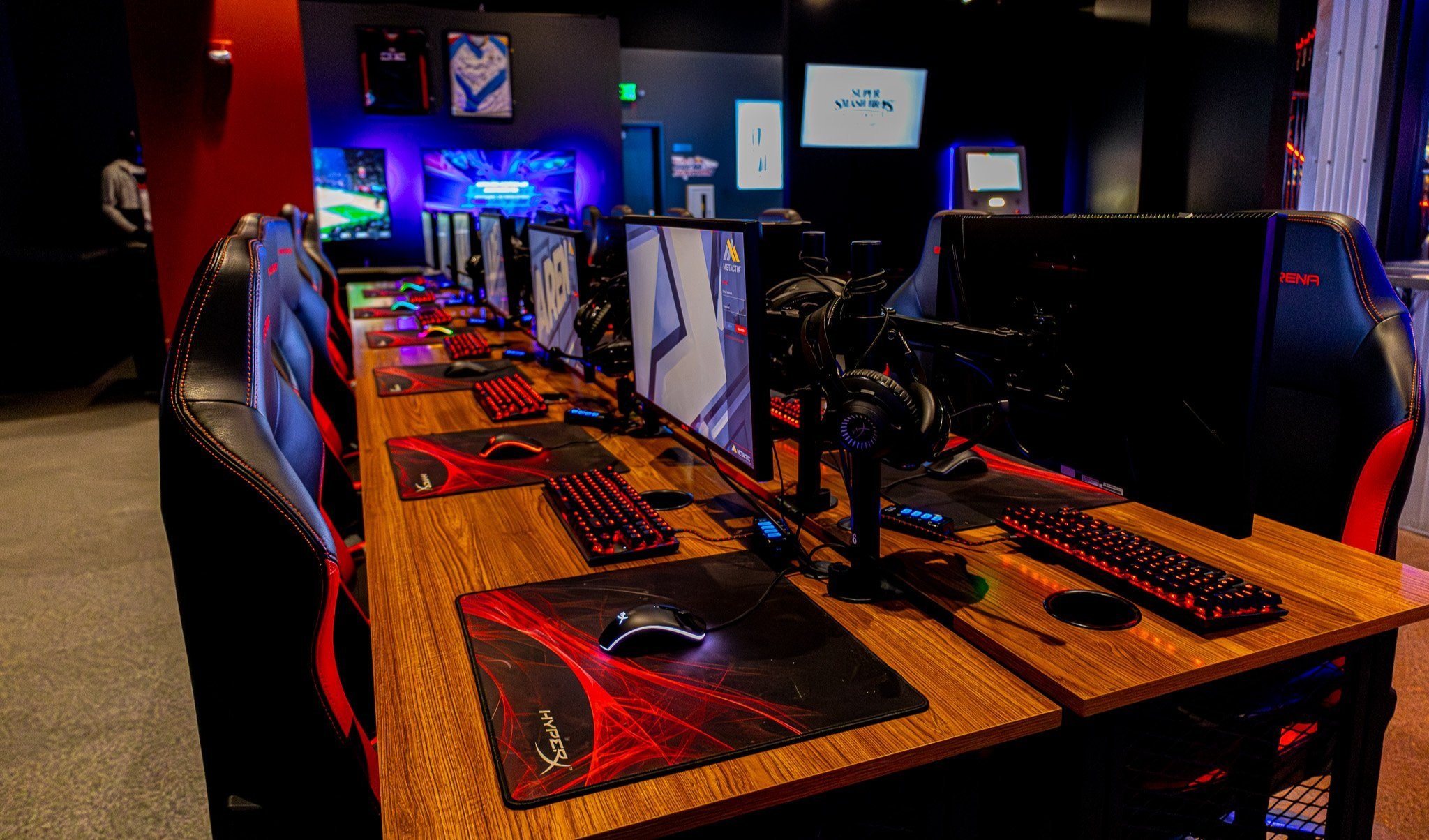The angled photograph showcases a meticulously arranged gaming cafe or PC bang, characterized by a sleek and glowing technological aesthetic. The room is set against a gray carpet and features a partially open black door to the left, revealing a maroon or red wall that provides a striking backdrop. Dominating the field are two long tables, each equipped with six high-end gaming stations. Each station comprises a black monitor with red illuminated keyboards and an assortment of LED-lit mice, the lighting colors varying from white to rainbow hues. Every setup also includes a black and red HyperX gaming mouse pad with the HyperX logo emblazoned in white.

The gaming chairs, possibly made from leather or eco-leather, also sport red accents harmonizing with the overall theme. In addition to these main tables, the room includes additional monitors in the far section, hinting at even more gaming setups. Some details like silver scaffolding and what appears to be an ATM machine add to the café's industrial charm.

A television between the monitors on the left displays "Smash Brothers Melee," further amplifying the gaming atmosphere. Despite the advanced setup, no gamers are present in the image; instead, headphones hang unused on their respective stations, waiting for the next session. The manikin or person in the back adds a touch of intrigue to the scene, completing the high-tech, immersive gaming environment typical of a Korean gaming room.